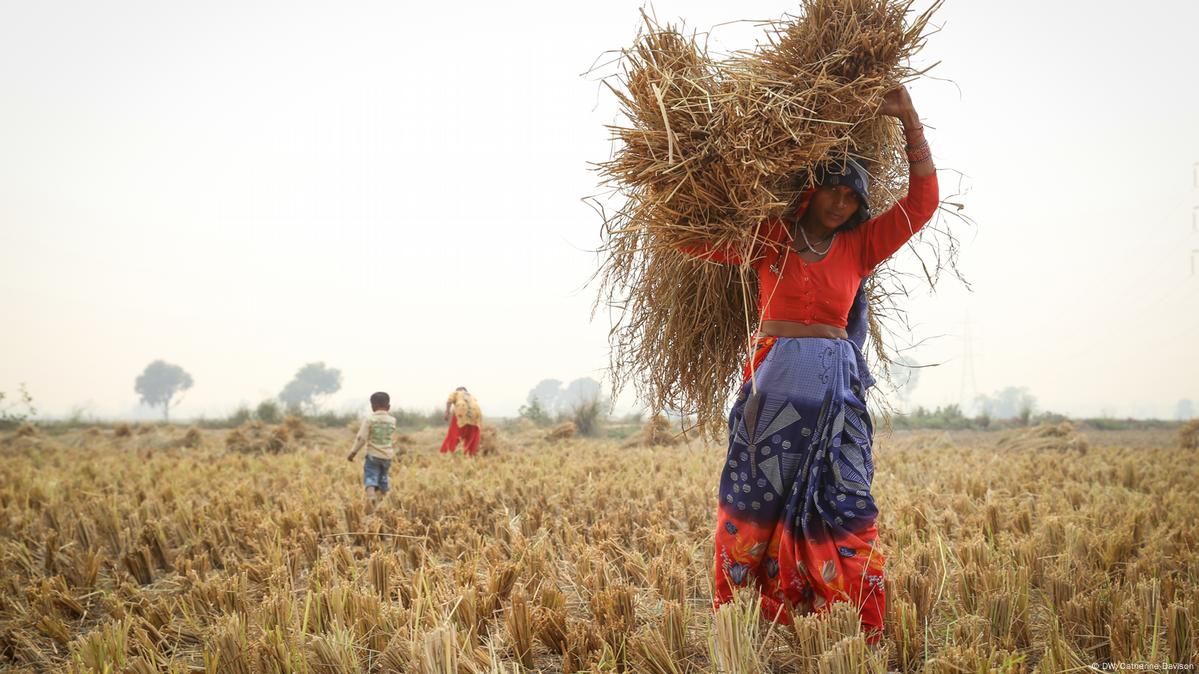The image depicts a young woman in an ethnic outfit working in a recently harvested field of grain, surrounded by clumps of light yellow weeds. She is dressed in a long sleeve orange shirt that reveals her midriff and a flowing skirt that transitions from blue to a darker blue with geometric patterns, ending in orange at the bottom. An orange and blue patterned scarf, matching her skirt, covers her head. She balances an armful of straw on her head and looks directly at the camera. In the background, a small child and an older individual, likely her family members, can be seen bent over and working in the same field. The overcast sky is light gray, and distant trees hint at an agricultural landscape. The image is credited to DW/Catherine Davison.